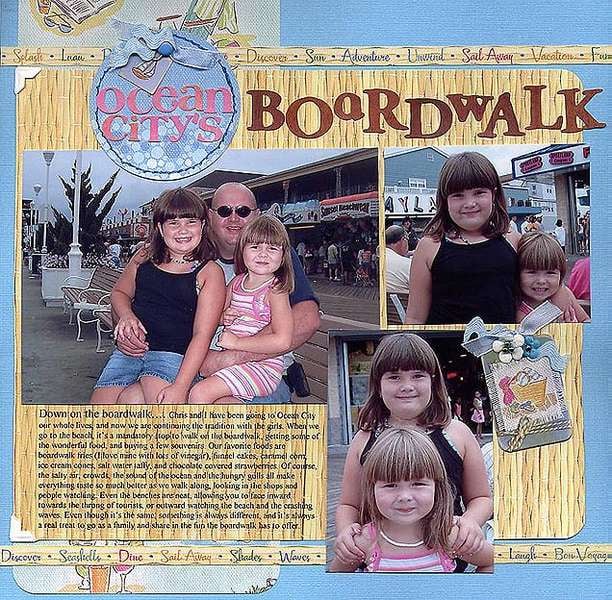The image features a detailed advertisement for Ocean City's Boardwalk, showcasing a visually striking collage against a textured blue background with an overlay of a square wood pattern. At the top center, the word "Boardwalk" is prominently displayed in large brown letters, while to the upper left, a circular emblem features the phrase "Ocean City's" in pink letters over a blue circle. Below this header, the collage includes three distinct photographs: 

1. On the left is a large photo of a bald middle-aged man in sunglasses, seated with two young girls on his lap. The girl on the left wears a navy blue tank top and jean shorts, while the one on the right is in a pink and white striped sleeveless dress. Behind them, a bustling crowd suggests they are at a lively gathering, potentially on the actual boardwalk, with a white and wood empty bench visible to the left.

2. To the right of this image is a smaller square photo featuring the same two girls standing side by side, arms around each other, with both gazing directly at the camera. They have straight brown hair, with the girl on the left possessing darker hair.

3. Below the smaller photo, another vertical rectangular picture shows the taller girl in the navy blue tank top standing protectively behind the shorter girl in the striped dress.

In the bottom left-hand corner, a block of text begins with "down on the boardwalk..." followed by approximately 15 lines of promotional description in a small black font, making it part of an elaborate advertisement for this seaside amusement destination.